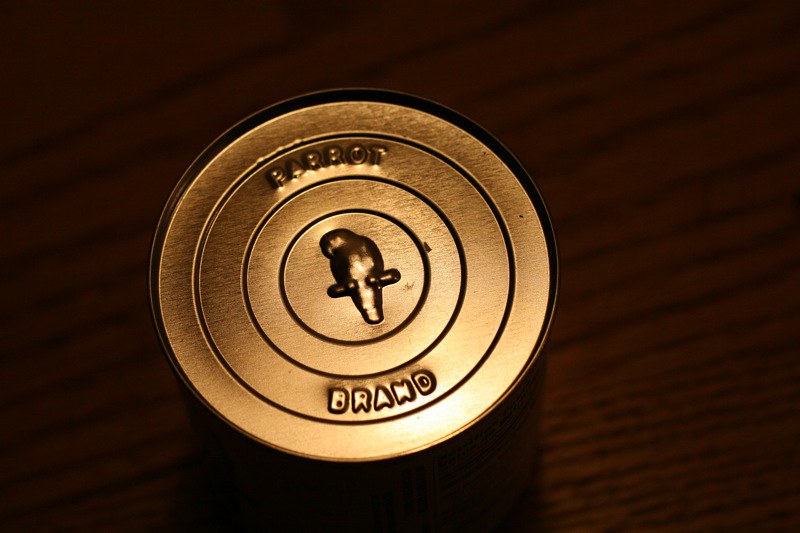This is a close-up photograph, taken in landscape orientation, capturing the top view of a vintage tin can. The image is slightly elevated, offering a perspective that looks down onto the can. At the top of the can, the word "Parrot" is prominently etched into the metal, while at the bottom, the word "Brand" is similarly inscribed. Centrally located on the face of the can is a detailed depiction of a parrot, crafted in vibrant hues that stand out against the metallic background. The can is resting on a table made of dark brown wood, which features pronounced grain patterns running diagonally from the lower left to the upper right corner, adding texture and contrast to the composition.